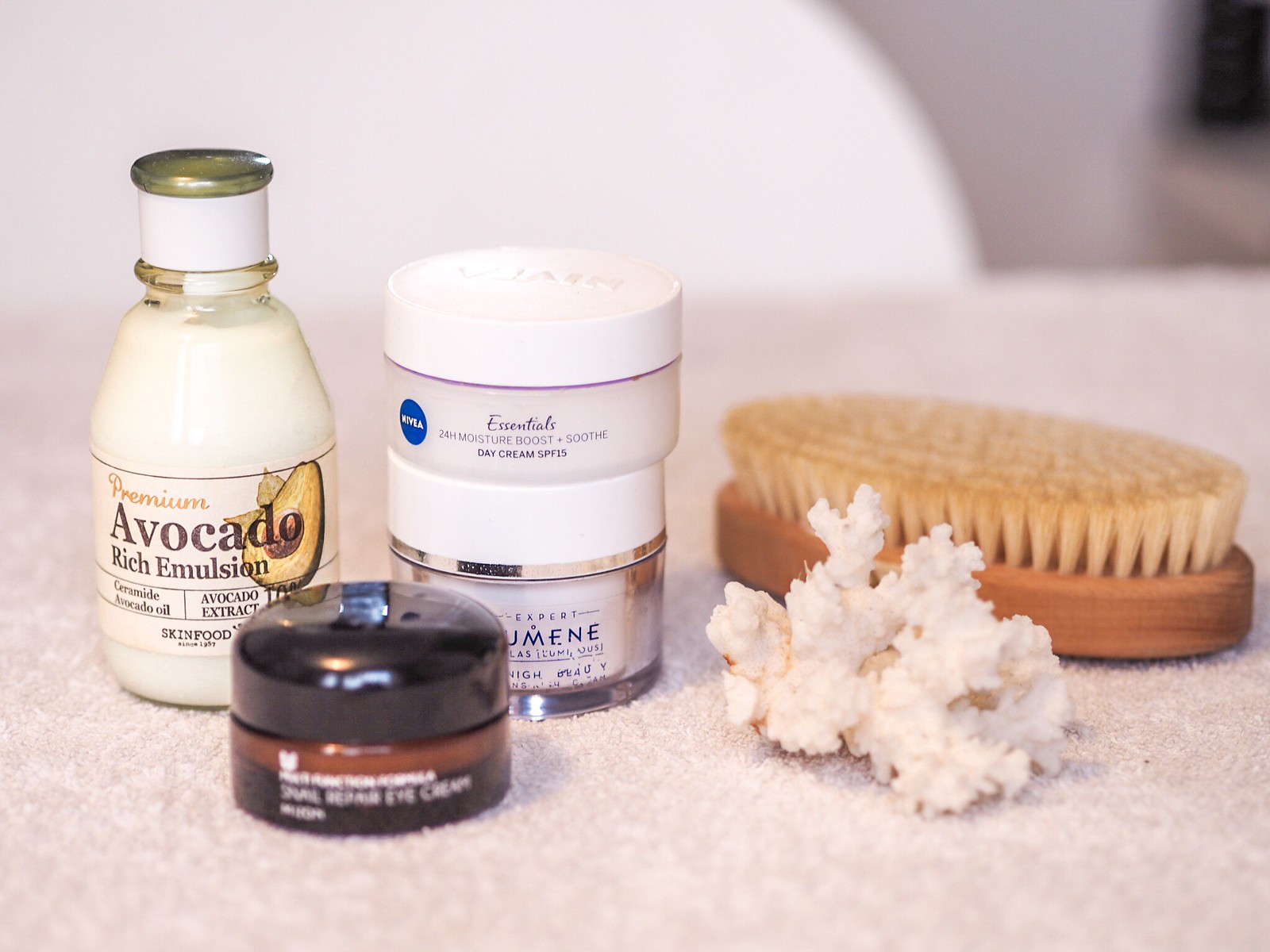The photograph showcases an array of beauty products arranged neatly on a soft, tan-colored towel. Dominating the composition is an oval-shaped brush with a wooden handle, resembling bamboo, with white, tan bristles adding a touch of natural elegance. In front of the brush sits a white piece of coral, serving as a decorative accent.

To the left of the coral are two jars of cream. The first jar is translucent at the bottom, topped with a white lid, while the second jar is opaque with a white lid, labeled "Nivea Essentials 24-Hour Moisture Boost + Soothe Day Cream SPF 15."

In the bottom left corner of the frame, a two-tone brown jar can be seen, labeled "Snail Repair Eye Cream." Adjacent to this jar, on the far left, is a white bottle, likely made of glass, with a green stopper. The bottle bears a white label that reads "Premium Avocado Rich Emulsion, Ceramide, Avocado Oil, Avocado Extract."

Overall, the arrangement exudes a sense of luxury and care, with each item thoughtfully placed to create an aesthetically pleasing display.